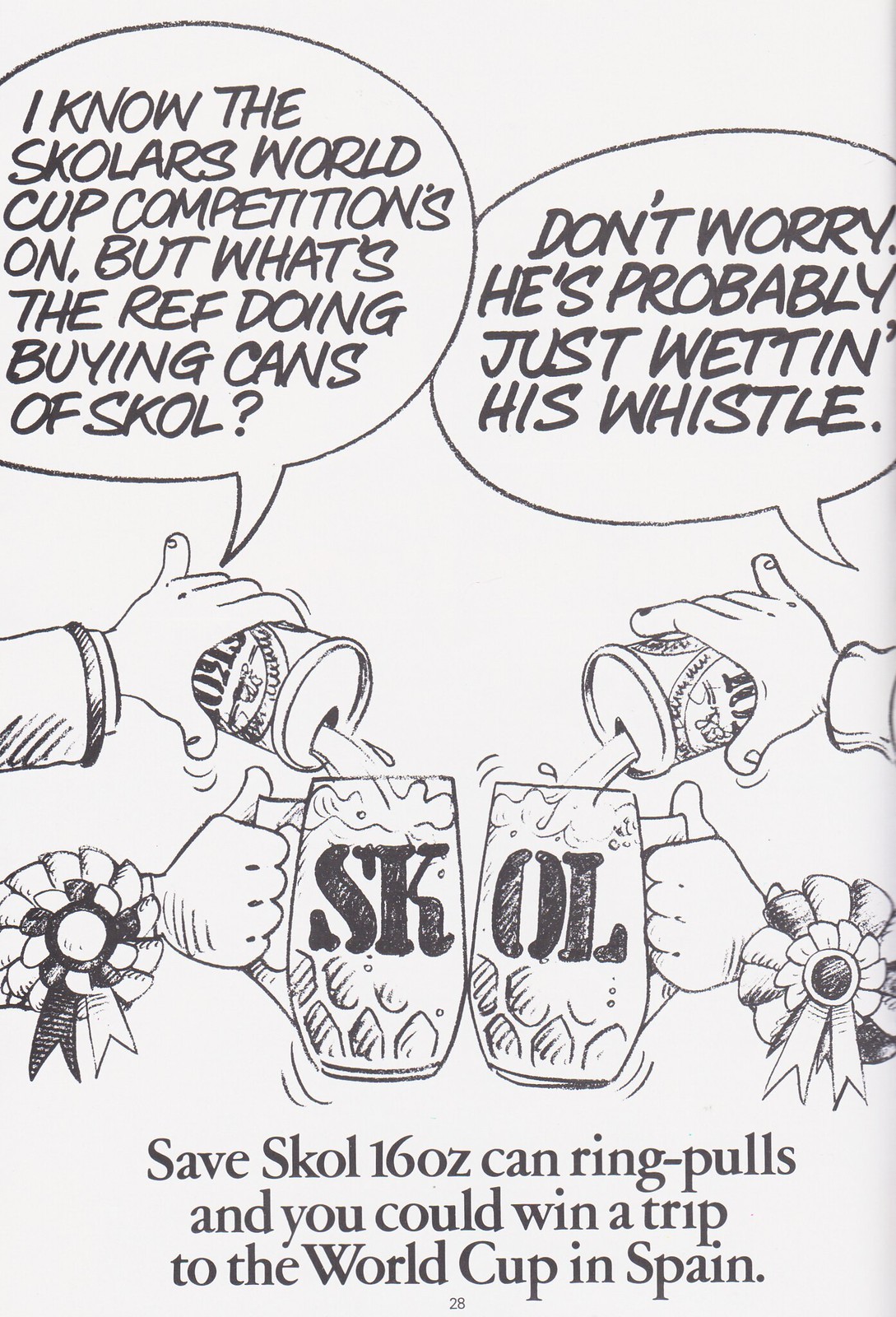This vertically aligned, black-and-white image resembles a single-panel comic strip. It features four hands: two from the left and two from the right. The two top hands pour canned drinks labeled "SKOL" into glass mugs held by the bottom hands, which also grasp the mug handles. The mugs, marked with large "SK" on the left and "OL" on the right, touch to spell out "SKOL." Additionally, each top hand wears a ribbon on its wrist, suggesting an award. Above the hands are two speech bubbles. The left bubble reads, "I know the Scholar's World Cup competition's on, but what's the ref doing buying cans of SKOL?" To which the right bubble responds, "Don't worry, he's probably just wetting his whistle." At the bottom of the image, a caption states, "Save SKOL 16-ounce can ring pulls and you could win a trip to the World Cup in Spain."